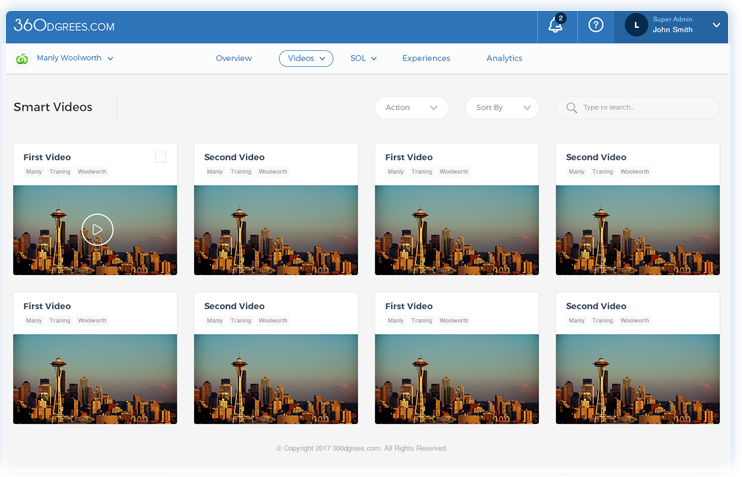The screenshot captures a computer screen displaying a webpage from 360degrees.com. In the top right corner, a blue border displays the website's name, alongside a notification bell indicating two new notifications, a circle with a question mark, and a drop-down menu labeled “Super Admin John Smith” featuring a black circle with an "L" inside it. Below this header, a white border frames the content with a drop-down menu on the left labeled “Manly Woolworth.” Next to it, there are navigation options including "overview," "videos" (highlighted with a circle), "SOL," "experiences," and "analytics."

The main section of the screen showcases the title “Smart Videos” in the upper left corner. Adjacent to the title, on the right, are two drop-down menus labeled “Action” and “Sort By,” followed by a search bar that prompts with "Type to Search."

The center of the screen features a grid of eight video thumbnails, arranged in two rows of four. Each thumbnail displays an identical image: a sky background with the Seattle Space Needle on the left and smaller skyscrapers on the right. The video titles on the top row are labeled sequentially as “first video,” “second video,” “first video,” and “second video.” The bottom row mirrors this labeling with the same titles: “first video,” “second video,” “first video,” and “second video.”